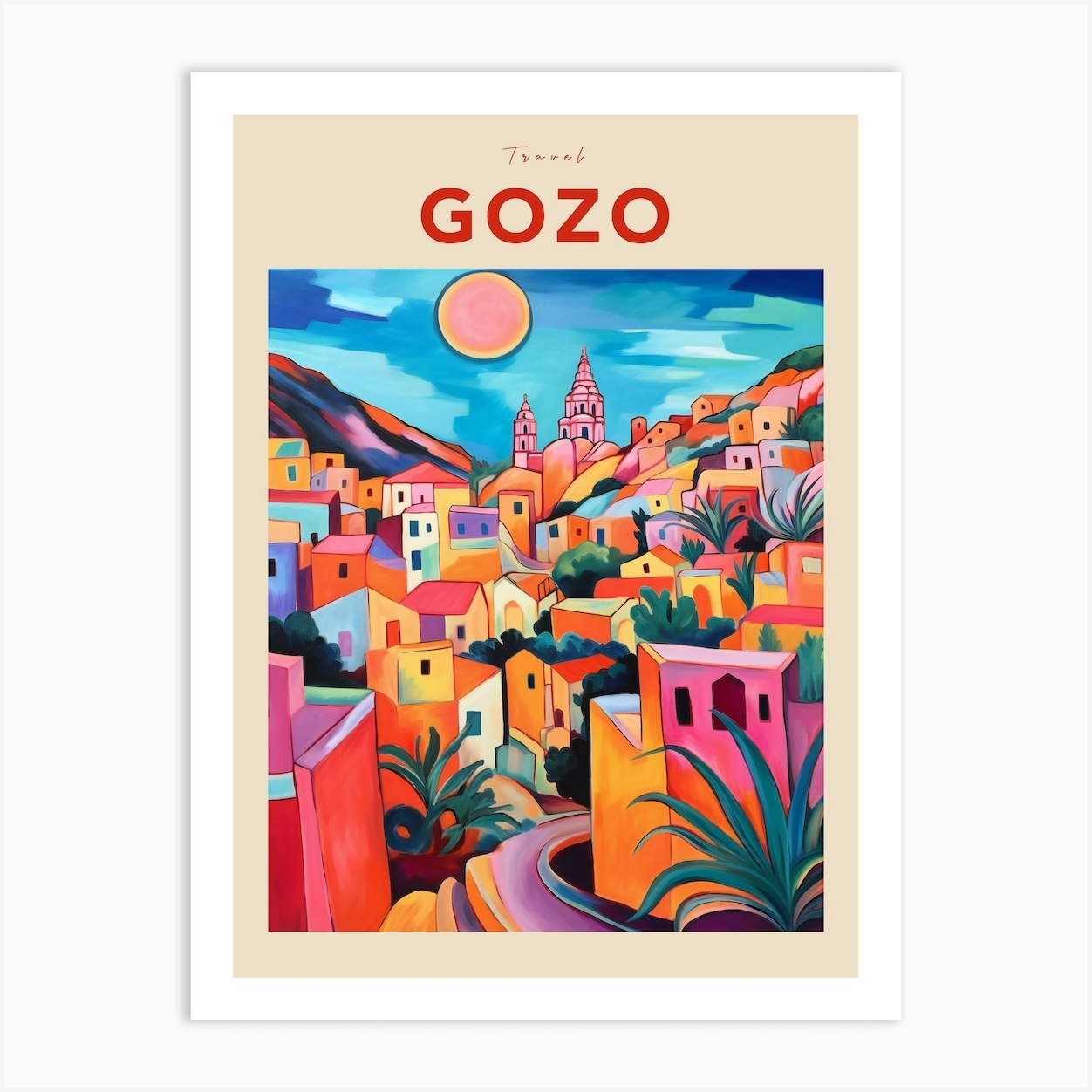The image is a travel poster hanging on a white wall, framed by a white border with a subtle drop shadow. The poster itself has a large light beige border, especially thick at the top where "travel" is written in small red cursive text. Below that, in large, bold, sans serif red letters, it reads "GOZO," G-O-Z-O. The centerpiece of the poster is a vibrant, minimalist illustration done in a style reminiscent of Cezanne. The artwork depicts a colorful city situated in a valley, with buildings in hues of orange, yellow, pink, purple, and red. Interspersed among the buildings are green plants and trees, creating a rich, lively scene. A street runs into the city, leading the eye toward a distant church perched atop a hill. The sky above the city is a combination of blue and cloudy, with a setting sun that is orange in the center, fading to yellow around the edges. The overall effect is a dynamic and warm portrayal of Gozo, inviting the viewer to explore the picturesque location.